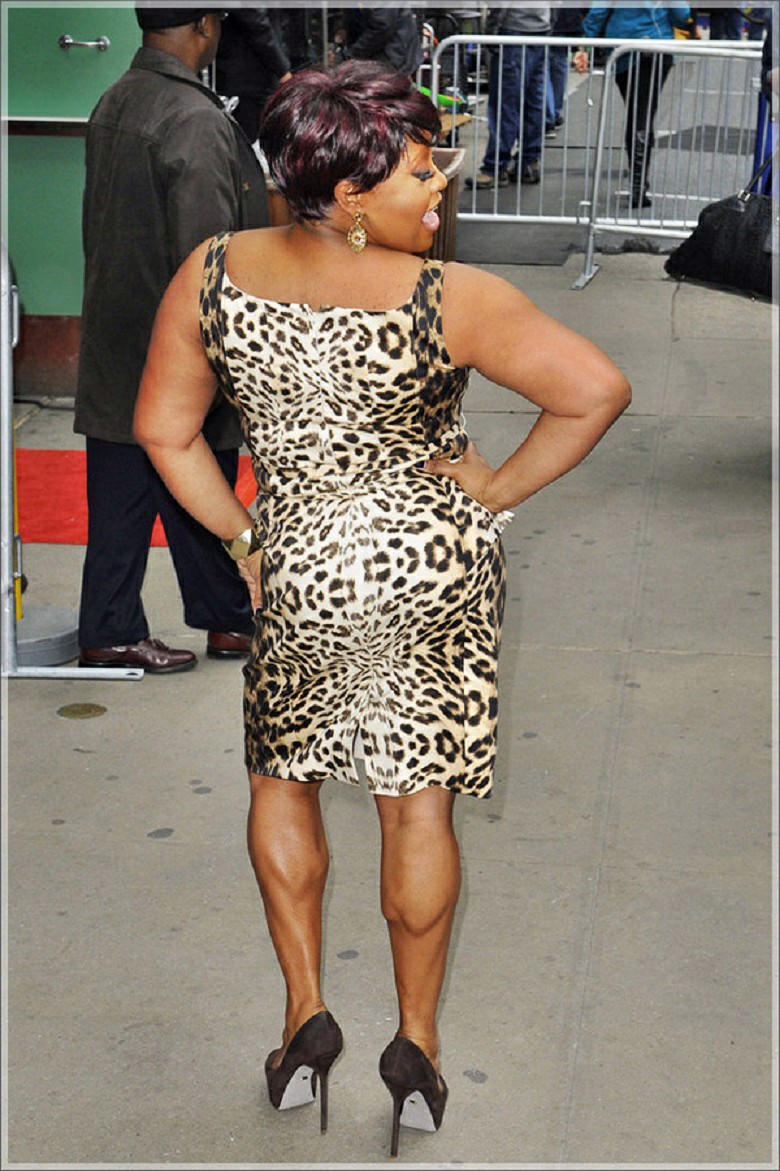In this vibrant outdoor scene, Sherry Shepherd is elegantly posing against the backdrop of a bustling event, likely a red carpet affair. She stands confidently on the sidewalk, her back turned to the camera while looking over her right shoulder, her mouth open as if she's in mid-conversation. Sherry is dressed in a striking sleeveless animal print dress—likely leopard or cheetah—that falls just above her knees, complemented by strappy high heels that accentuate the defined muscles in her calves. Her short hair, a mix of black and red or purple hues, frames her oval earrings and adds a bold touch to her look. She accessorizes with a metal bracelet and eyelash extensions, enhancing her glamorous appearance. With one hand stylishly perched on her hip, Sherry's pose encapsulates confidence and grace. In the background, a gentleman dressed in a dark coat and slacks stands near the entrance of a red carpet, behind silver barricades set up to manage the crowd. The scene, marked by daylight, captures the essence of a high-profile public event.